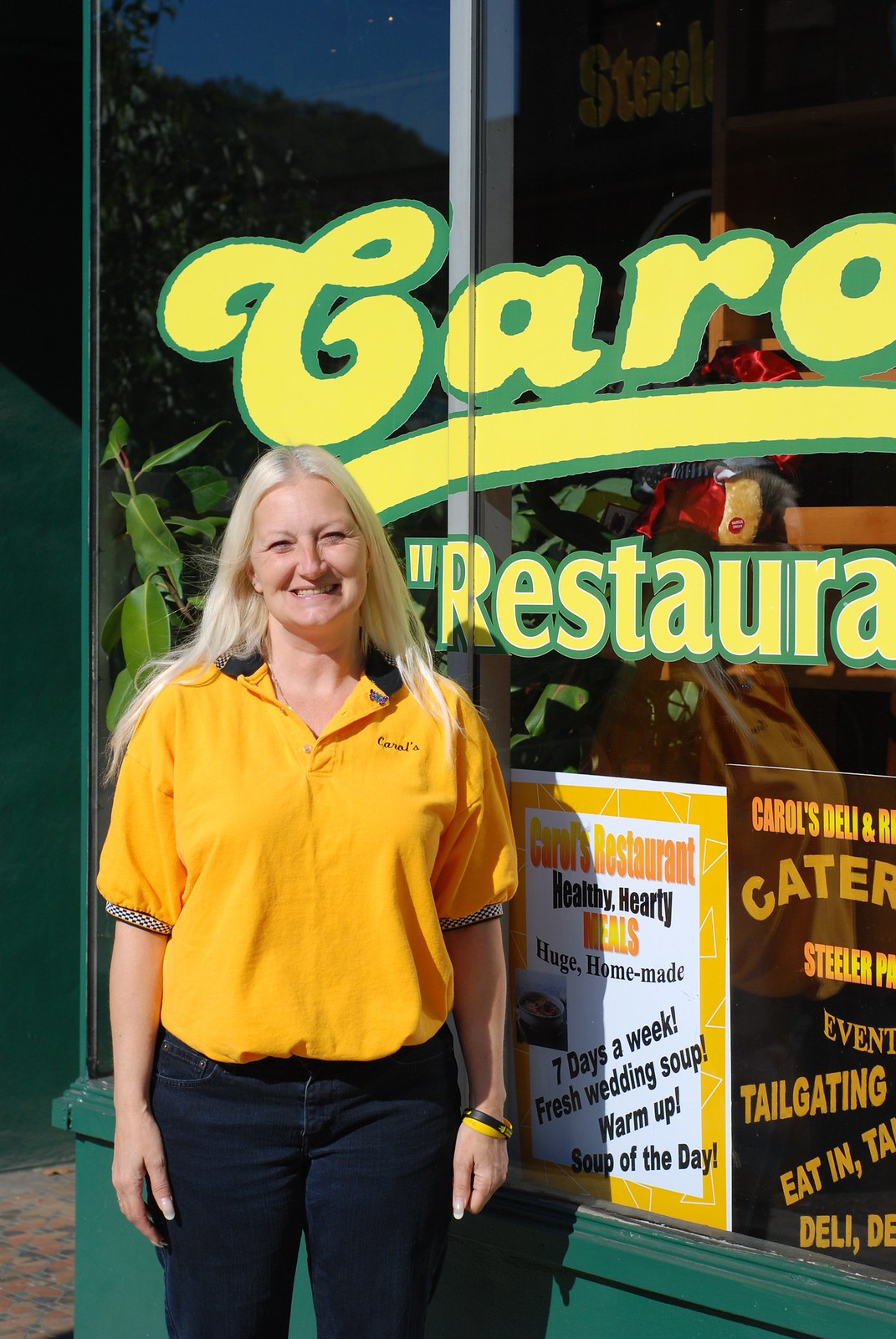In this outdoor daytime photograph, a smiling blonde woman stands in front of a restaurant confidently. Her outfit consists of an orange polo shirt with black slacks, and the logo C-A-R-A-T's is visible on her shirt. The woman, possibly an employee, stands with a bracelet on her wrist. She poses in front of a plate glass window of "Carrows Restaurant," behind which various signs advertise the establishment's offerings. The window displays signs that read "Carrows Restaurant," promoting "Healthy, hearty meals, huge homemade dishes," available "seven days a week," featuring "fresh wedding soup, warm up, soup of the day." Additional advertisements on the side highlight services like "catering," "tailgating," "eat-in," and "takeout." A green plant can be seen peering over her shoulder, adding a touch of nature to the scene.